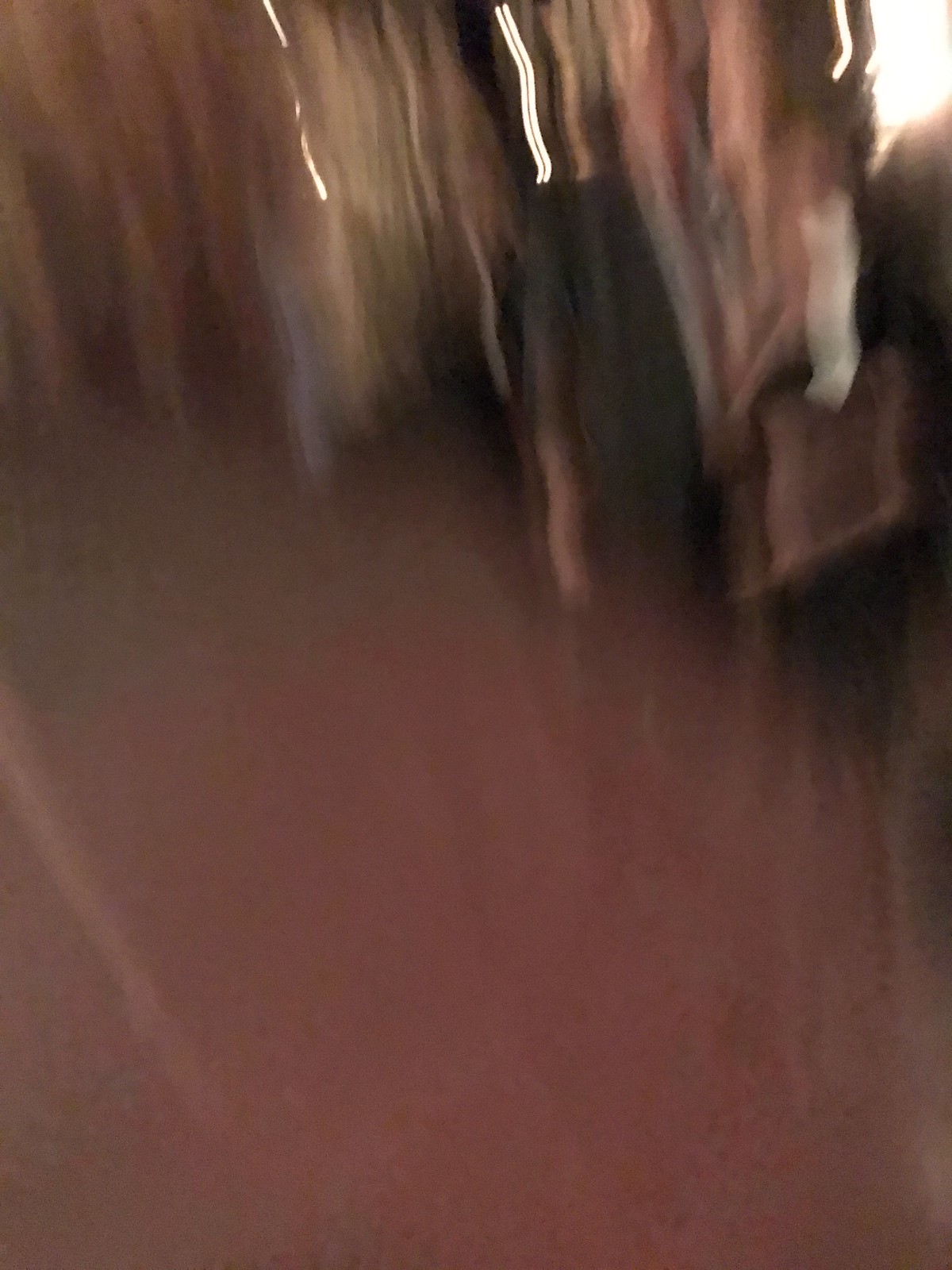The image appears to be an abstract, low-resolution photograph characterized by its blurriness and lack of focus. In the upper right corner, there's a noticeable white smear that stands out. Extending from the top of the photo down to its center are several light brown smears, giving the image a streaked appearance. Three prominent, hot white lines traverse the scene, resembling either flowing water or fabric caught in motion. The majority of the photo, around two-thirds, is dominated by a solid gray color, suggesting an underexposed or poorly lit ground. Additionally, there's a whitish smear across the lower right corner, which seems to emit a faint light, possibly adding a hint of illumination to the otherwise dim composition. Overall, the photograph carries an unintentionally abstract aesthetic due to its poor quality and indistinct subject matter.